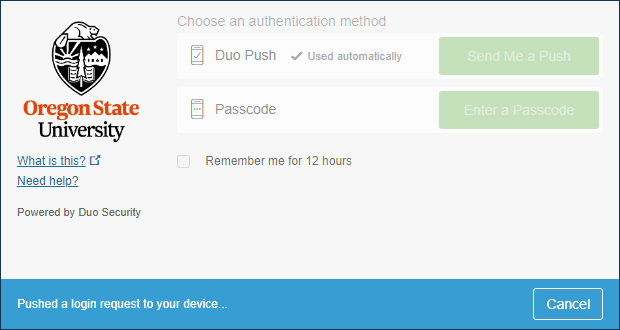The image features a prominent light blue box in the background, bordered by a black line. At the top of the box, there is a black heart icon. Below the heart, an illustration depicts various elements including a tree, sunshine, a cloud, a book, and what appears to be a beaver perched atop the book. The text "Oregon State" is written in bold orange letters, followed by "University" in black.

Further down, in blue text that is underlined, the caption "What is this?" appears, accompanied by an icon of a paper and pen. Nearby, another underlined text reads "Need help" with a smaller accompanying icon. 

The image is powered by Duo Security, as indicated by the text. At the center, the phrase "Choosing authentication method" is displayed. Below this, a white box offers two options: "Duo Push" with a checkbox stating "Use automatically", and "Passcode". A small box labeled "Remember me for 12 hours" is also present.

To the right, two buttons offer choices: "Send Me a Push" and "Enter a Passcode". At the bottom of the image, a bright blue box features the text "Push to log in requested to your device" in white. Finally, in the lower right corner, a blue box outlined in white with the word "Cancel" in white text completes the scene.